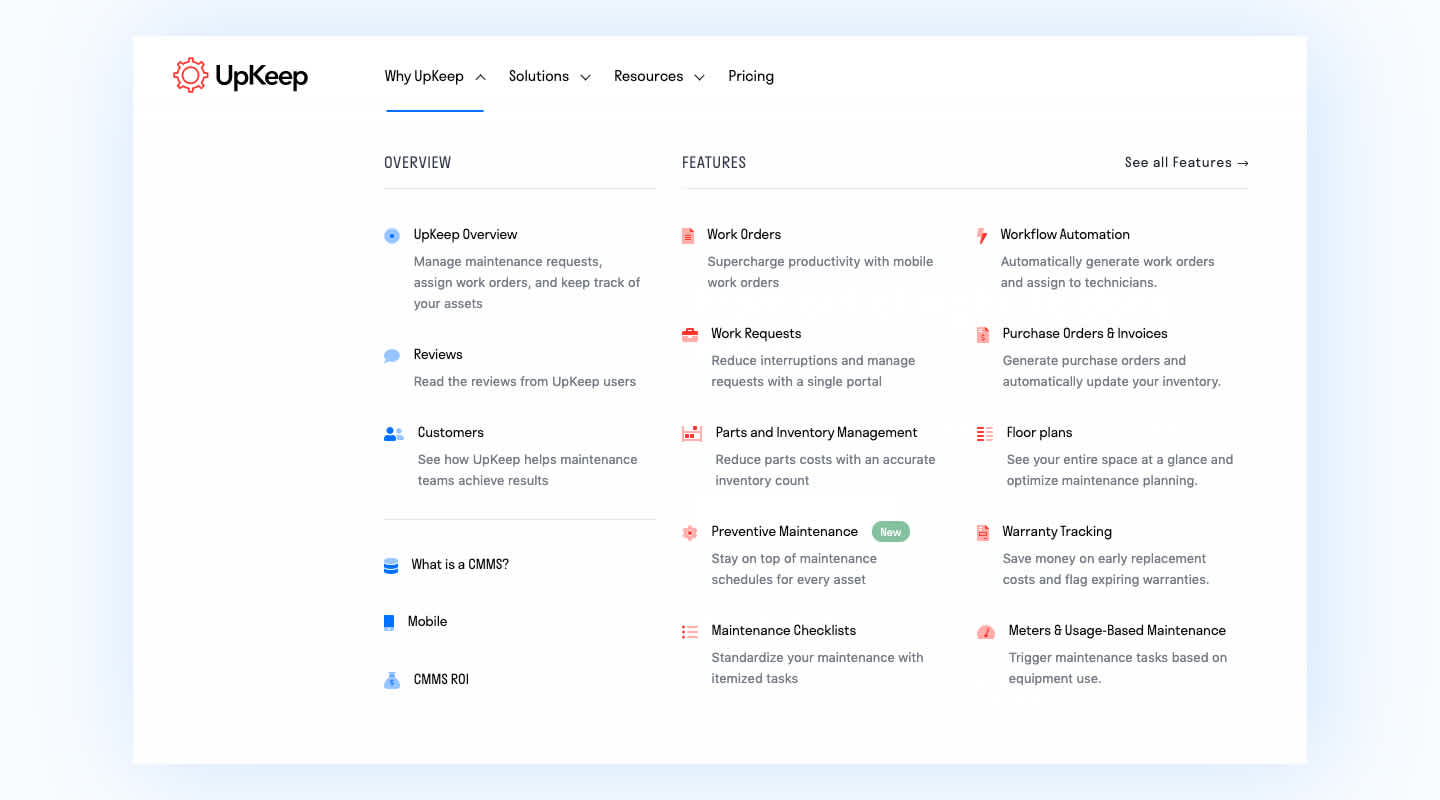This image portrays a detailed feature page from a website named "Upkeep." The page is primarily white, with a red gear icon and "Upkeep" displayed prominently in the upper left corner. At the top, a bold menu outlines sections including "Why Upkeep?", "Solutions," "Resources," and "Pricing." This specific page is under "Why Upkeep?" Below the menu, the "Overview" section includes subsections such as "Upkeep Overview" — where users can manage maintenance requests, assign work orders, and keep track of assets, "Reviews" — showcasing user feedback, and "Customers" — demonstrating how Upkeep benefits maintenance teams. Additionally, there's "Features," inviting users to "See All Features," with various capabilities highlighted: "Work Orders" to enhance productivity with mobile orders, "Work Requests" to manage through a single portal, "Parts and Inventory Management" to reduce costs with accurate counts, "Preventative Maintenance" to adhere to schedules, "Maintenance Checklists" to standardize tasks, "Workflow Automation" for auto-generating work orders, "Purchase Orders and Invoices" for inventory updates, "Floor Plans" for space optimization, "Warranty Tracking" for cost-saving on replacements, and "Meter and Usage-Based Maintenance" to trigger tasks by equipment use. The icons representing "Overview" are blue, while feature icons are red, giving a structured and vibrant look to the page.